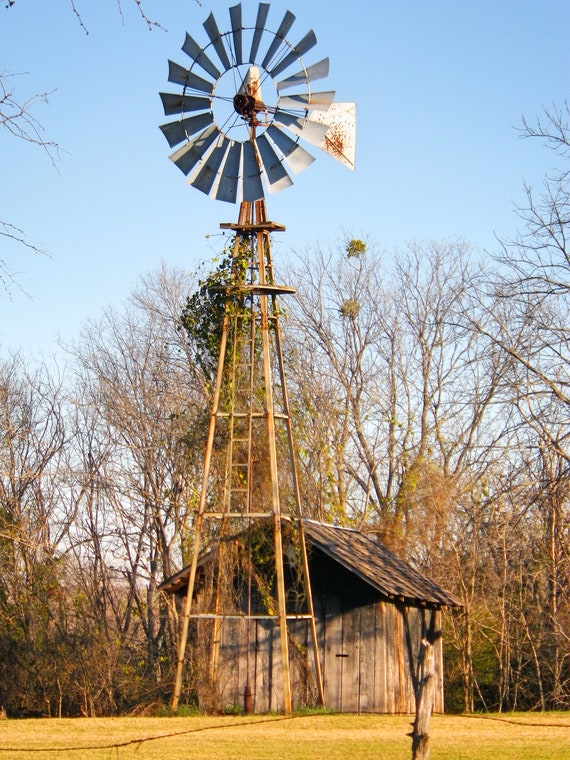The image captures a tall, slender windmill standing prominently in a field with weathered yellowish-green grass. The windmill has a triangular metal tower painted in a yellowish hue and features a circular rotor with rectangular blades, complete with a tail at the back for directional stability. A ladder runs up the side of the tower, adding to its rustic charm. Directly behind the windmill, there is a small wooden shed with weather-beaten brown planks and a triangular roof. Surrounding the shed and extending into the background are barren, thin-limbed trees, indicative of late autumn, with no leaves on their branches. Above, the sky is a clear, vibrant blue, completing the serene and slightly nostalgic pastoral scene.